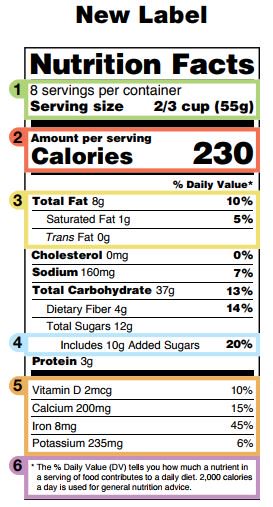This image depicts a nutrition facts label with a modern design marked as the "new label" at the top. The label is predominantly white, featuring black text to present the nutritional information. Key areas of the label are encircled and color-coded with numbers for emphasis and clarity. 

1. A green circle highlights "Servings per container," indicating its importance.
2. Calories are prominently displayed in red to draw immediate attention.
3. "Total fat" is marked with a yellow circle, underlining its content.
4. A blue circle encloses "Includes added sugars," stressing its nutritional significance.
5. Vitamins and minerals are encircled in orange, emphasizing their presence.
6. Finally, the "Explanation of the daily value" is surrounded by a purple circle, providing context for understanding the nutritional data.

This methodical color-coding and numbering enhance readability and help users quickly locate crucial nutritional information.